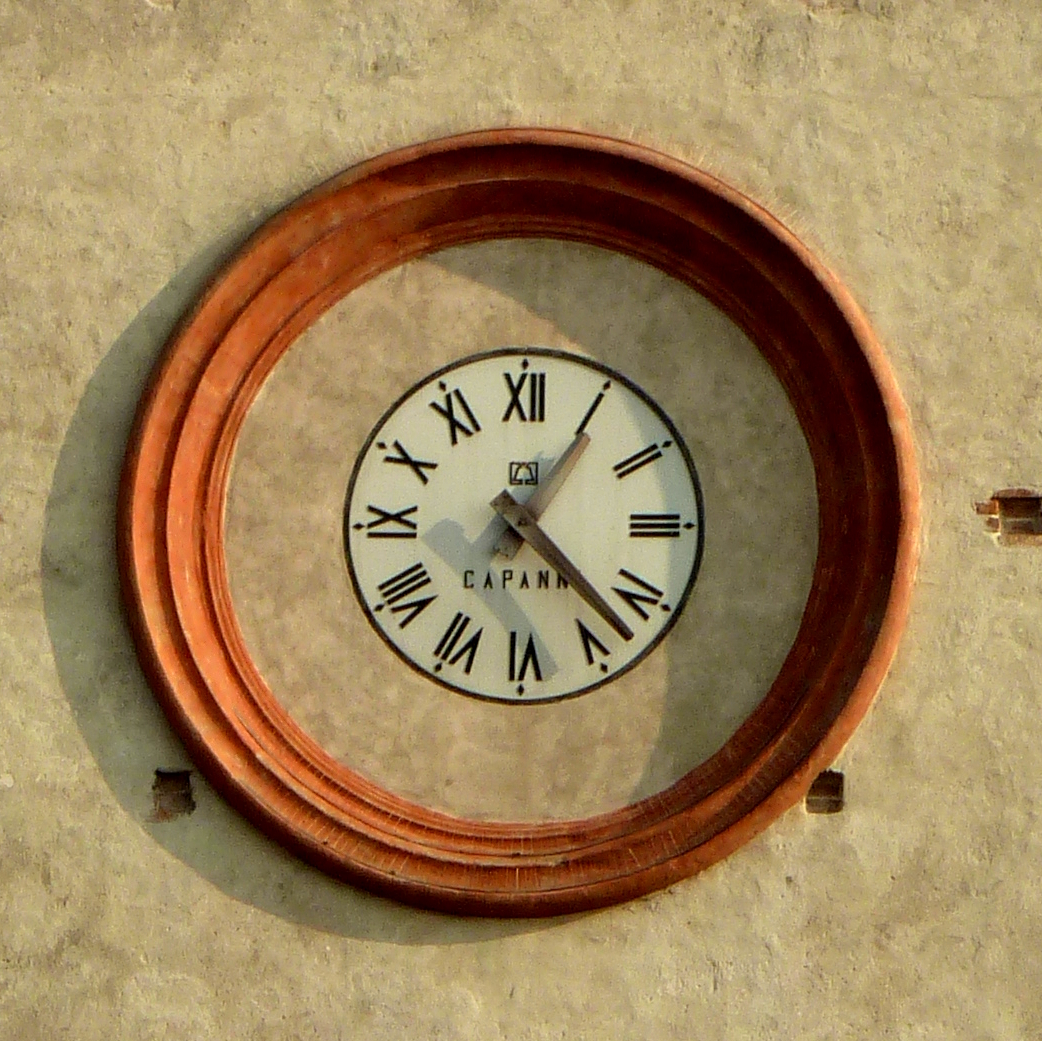Image Caption:

In the image, there is a detailed clock face with ornate features. The clock shows the hour hand perfectly aligned with a prominent marker, while the minute hand points between numerical indicators I, B, and V. Prominent markings resembling cat paw prints spell out "CAPANNA" around the clock's face. Above the ruby-colored numerals, diamond-shaped embellishments add a touch of elegance. The clock's center is encircled by a stone wall, revealing glimpses of brickwork through small gaps, reminiscent of a historical façade. The exterior of the clock includes multiple red clay circles, arranged concentrically, with lines intersecting them, enhancing the intricate design. The clock is well-illuminated on both the right and left sides, casting a bright white light, while the back remains predominantly white. However, the center right of the clock face is cloaked in shadow, adding depth to the visual composition.